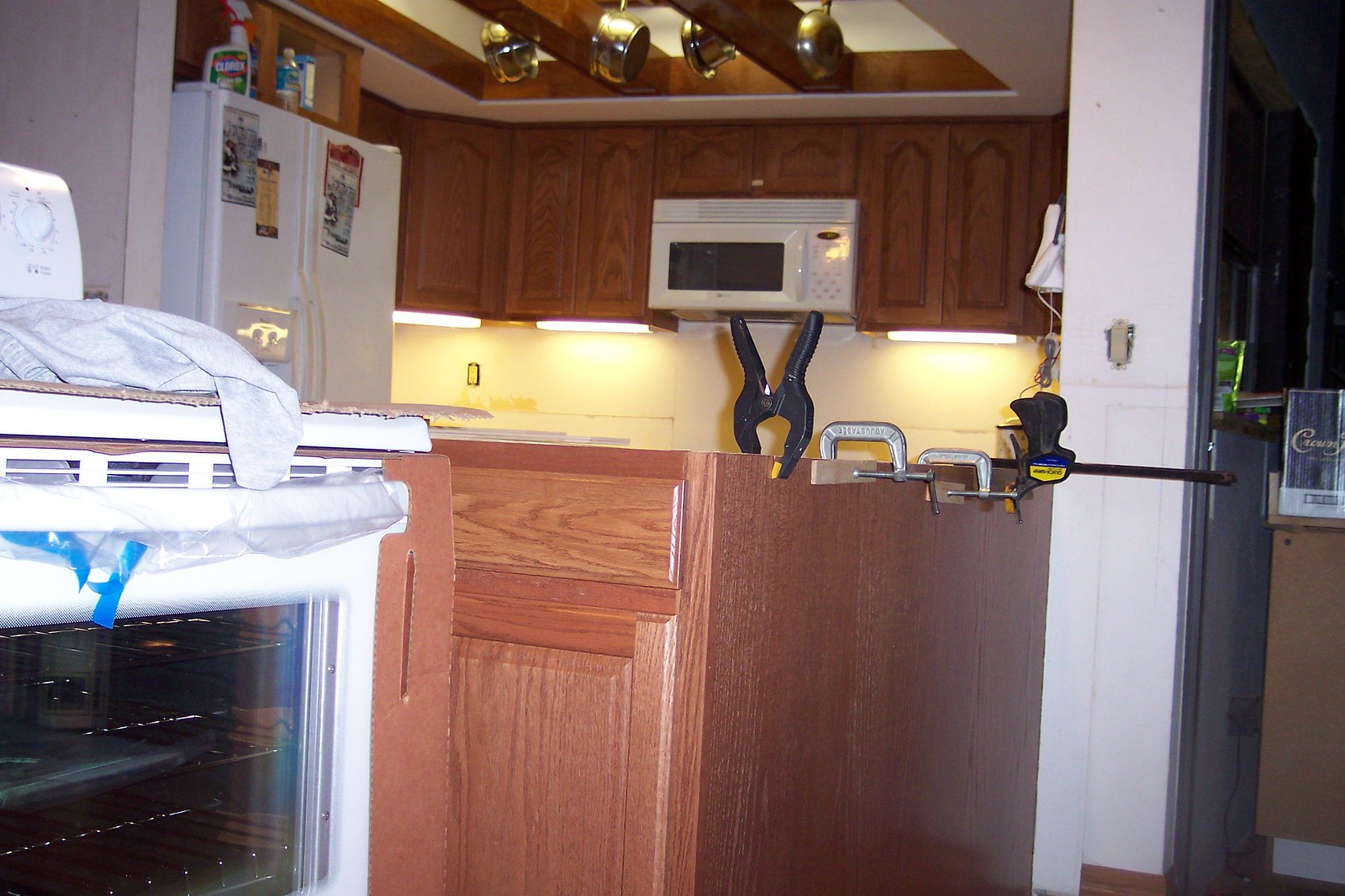A detailed image of a kitchen under renovation reveals several elements in the process of being updated. On the left-hand side in the foreground, a brand new, white oven still wrapped in protective plastic and cardboard suggests recent delivery. The plastic remains particularly noticeable on the oven handle. Behind the oven, a light tan cabinet frame is visible, intricately clamped together indicating it has been glued and is currently setting.

In the top right-hand corner of the image, a refrigerator partially appears, adorned with three magnets and a prominent blue and yellow UPS sticker. Atop the refrigerator, there's a spray bottle of Clorox bleach cleaner, identifiable by its white, red, and green color scheme. Additionally, open cabinets above the refrigerator house various bottles, hinting at an ongoing organizational effort.

The top portion of the image features a ceiling-mounted rack holding a variety of pots and pans, framed by a wooden border, which might be mistaken for a skylight at first glance. Surrounding the kitchen, cabinets line the upper walls, with a dedicated inlet space for a small microwave, further emphasizing the home's state of transition.

On the far right side of the picture, a white column stands out, seemingly constructed to conceal infrastructural elements. The overall scene depicts a kitchen in the remodeling stages, with evident progress toward completion but with many components still awaiting final placement.